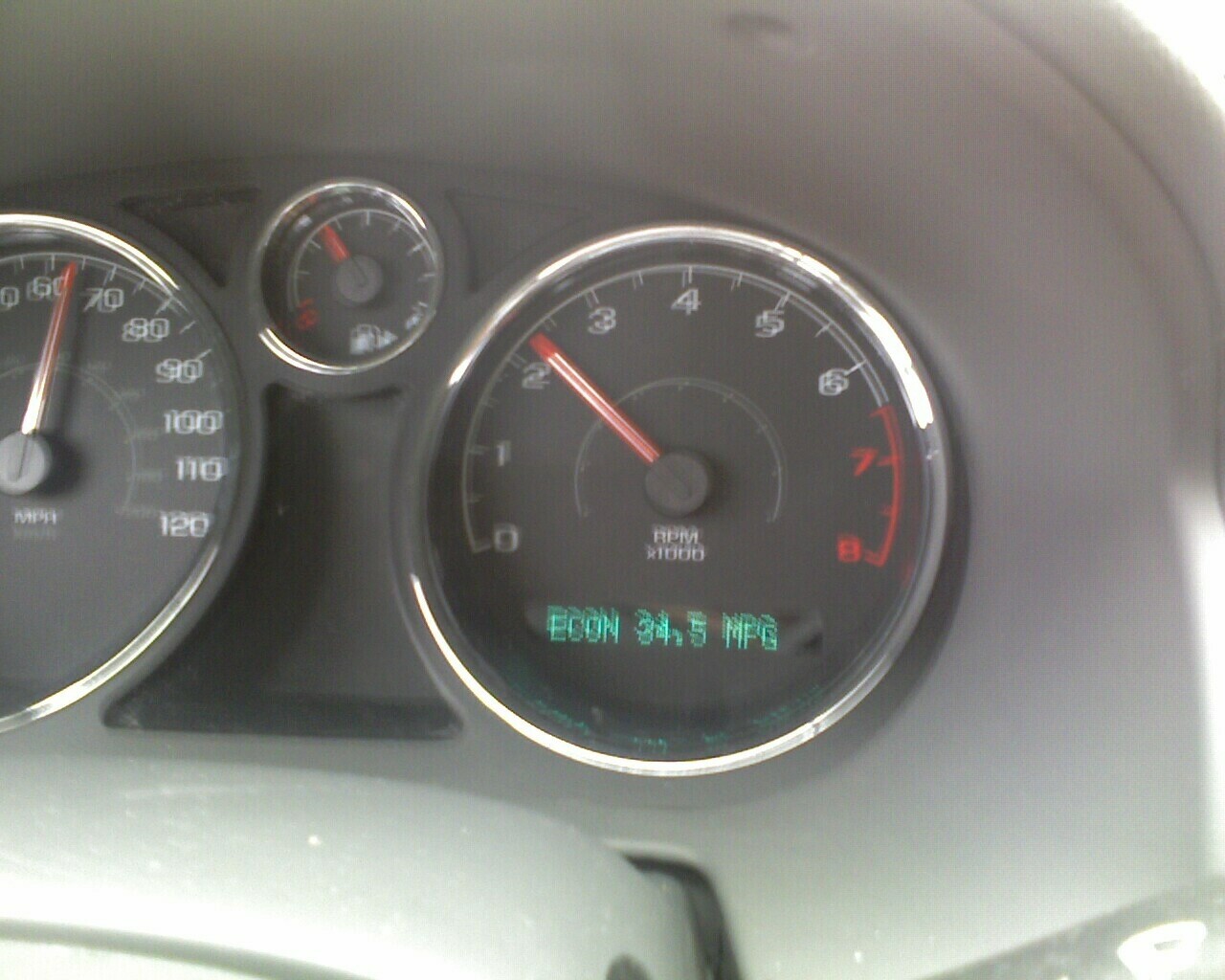This image, taken from inside a vehicle, showcases a detailed view of the car's dark gray dashboard, which is slightly blurry and grainy due to poor lighting. Front and center is the RPM meter, its black dial encircled with chrome and displaying white numbers that transition to red between the 7,000 and 8,000 RPM marks. The needle of the RPM gauge is orange and currently points just above 2,000 RPM. Beneath this gauge, a digital readout illuminated in green reads "ECON 34.5 MPG." The gas gauge, smaller than the others, sits in the center and shows a bit over a third of a tank remaining. To the left, partially cut off, is the speedometer indicating nearly 65 miles per hour. Each gauge is meticulously detailed with black dials, white lettering, and chrome outlines, contributing to the dashboard's cohesive and functional design.